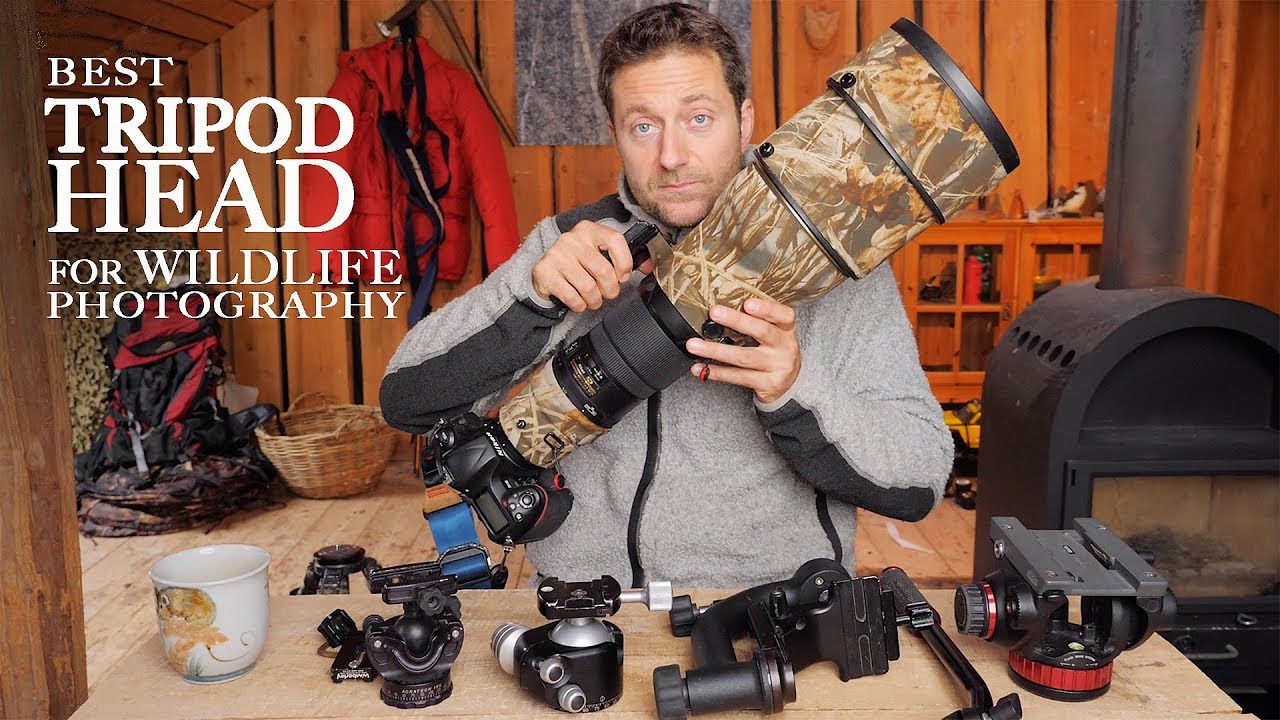In the image, designed as a thumbnail for a YouTube video titled "Best Tripod Head for Wildlife Photography," a man, who appears to be an expert in photography, is prominently featured. He is of Caucasian descent with brown hair and blue eyes, and he's clad in a light gray and dark gray fuzzy zip-up sweatshirt accented with black details. His attire suggests he’s dressed warmly, fitting the rustic setting that includes a wood-burning stove and wood-paneled walls, resembling a cozy cabin.

The man is holding a professional digital camera equipped with an enormous, camouflage-patterned zoom lens, approximately two feet long and about eight inches thick—ideal for wildlife photography. His facial expression appears somewhat disengaged as he poses with the camera.

In front of him, on a beige-colored table, lie multiple tripod heads of varying sizes, laid out for comparison. The largest tripod head to the right features a gray mounting track with black dials accented by red rims. The background is detailed with an orange wall, a red jacket hanging, and a brown basket on the floor, further enhancing the warm, woodsy atmosphere of the indoor setting.